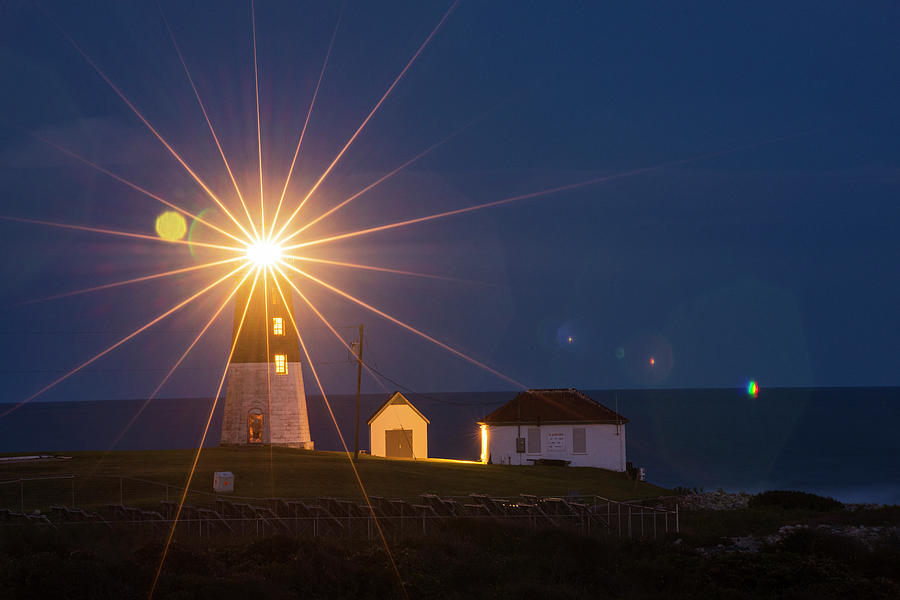This nighttime scene depicts a pristine lighthouse, possibly digitally altered or AI-generated, set against a dramatic dark blue sky and ocean. The lighthouse, characterized by its white brick base and darker painted upper section, is slightly off-center to the left with its bright, white-yellow light casting sharp, sun-like rays that dominate the upper half of the image. The structure features vertically-aligned windows illuminated in amber and white hues, and a doorway where a figure possibly stands.

In the foreground on the lower left, there's a dark green hillside with a rocky outcropping to the right, and a chain-link fenced area enclosing several slanted solar panels. To the right of the lighthouse sits a small white shed with a steeply pitched roof and a gray door. Adjacent to this is a larger white house featuring two windows, a brown roof, and an exterior adorned with a gray electrical box. The grassy terrain surrounding these buildings is vibrant with green hues, accented by scattered gray rocks and the gentle glow of the moon low in the sky to the left.